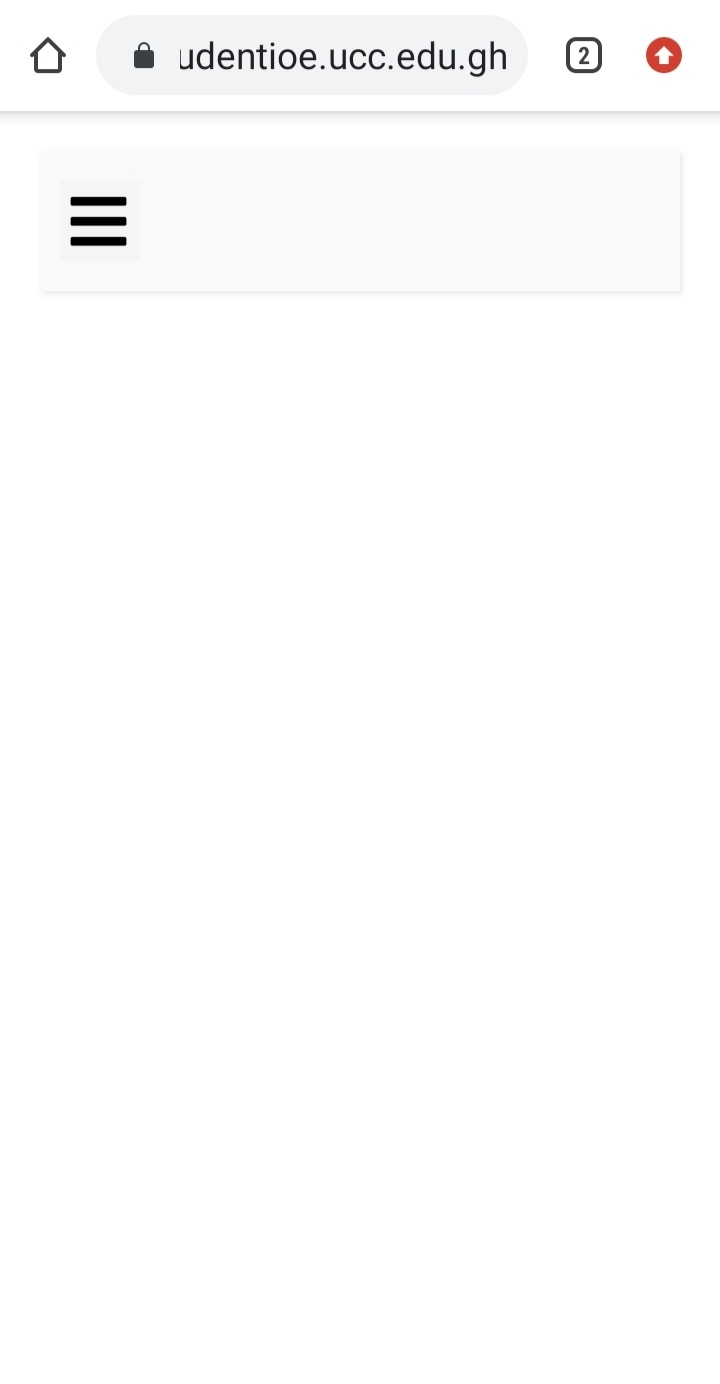This image is a screenshot of a website interface featuring a minimalist design with a predominantly white background. At the top of the image, there is a small black outline of a house icon. Directly to the right, a light gray address bar is visible, which includes a black padlock graphic symbolizing a secure connection. The address bar displays a partial URL: "...UDENTIOE.UCC.EDU.GH."

Next to the address bar, there is a black-outlined square with a white background, containing the number "2" in the center. Slightly further right, a dark red circle draws attention with its bold white arrow inside.

Below this section, a thin horizontal gray line spans the width of the image, demarcating the upper elements from the main body of the website. Underneath this line, the background remains white.

Further down, a light gray rectangular button is positioned, featuring three horizontal black lines on its left side. These lines are equally spaced and uniform in length, representing a typical menu icon.